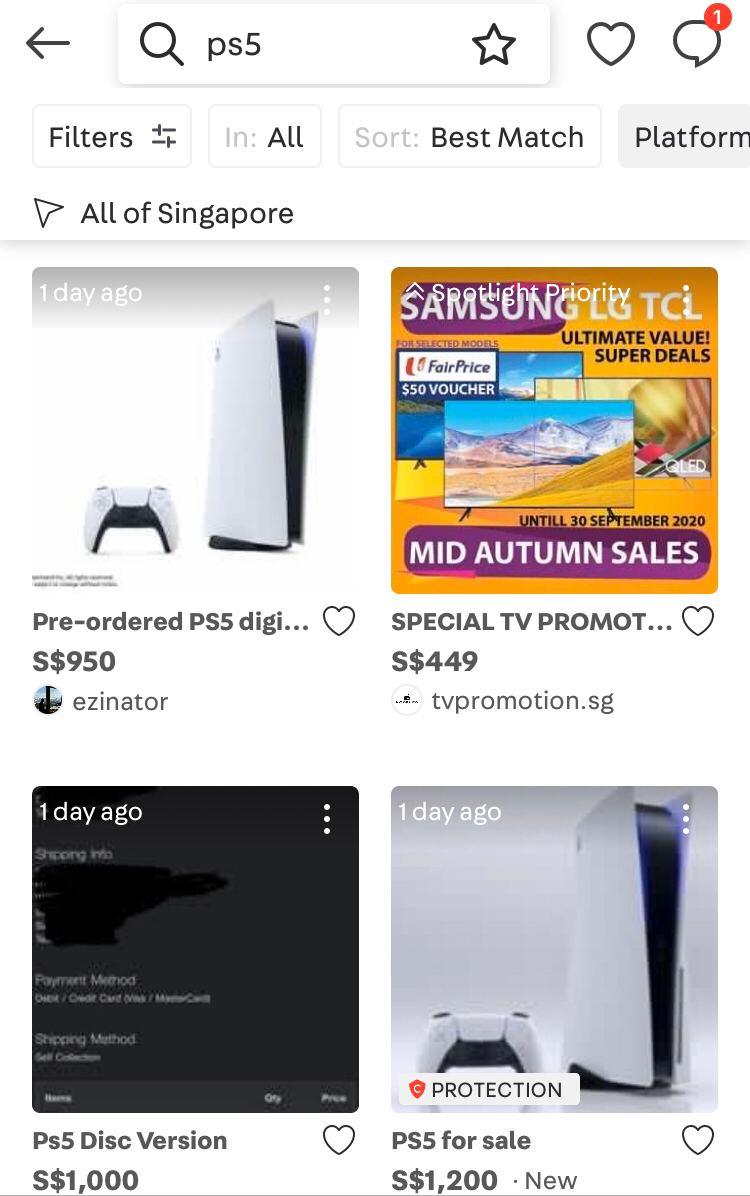The screenshot was captured from a mobile device and features a white-themed interface. In the upper left corner, a back arrow is visible, offering a navigation option. Centrally at the top of the screen is a search bar, containing the term "PS5" and accompanied by a magnifying glass icon to its left. To the right of the search bar, there are two icons: a heart-shaped icon and a text bubble icon displaying a red circle with the number "1" inside it.

In the main section of the screen, there are four thumbnail images organized into two rows and two columns. The first thumbnail, located at the upper left, displays a game controller and a game box in white and black hues. Adjacent to it, in the upper right, is an image characterized by a yellow and purple color scheme, advertising mid-autumn sales. The third thumbnail, positioned at the lower left, features a dark, grayed-out aesthetic with the words "One Day Ago" superimposed on it. There is no description provided for the fourth image in the lower right, indicating it may not have been fully visible in the screenshot.